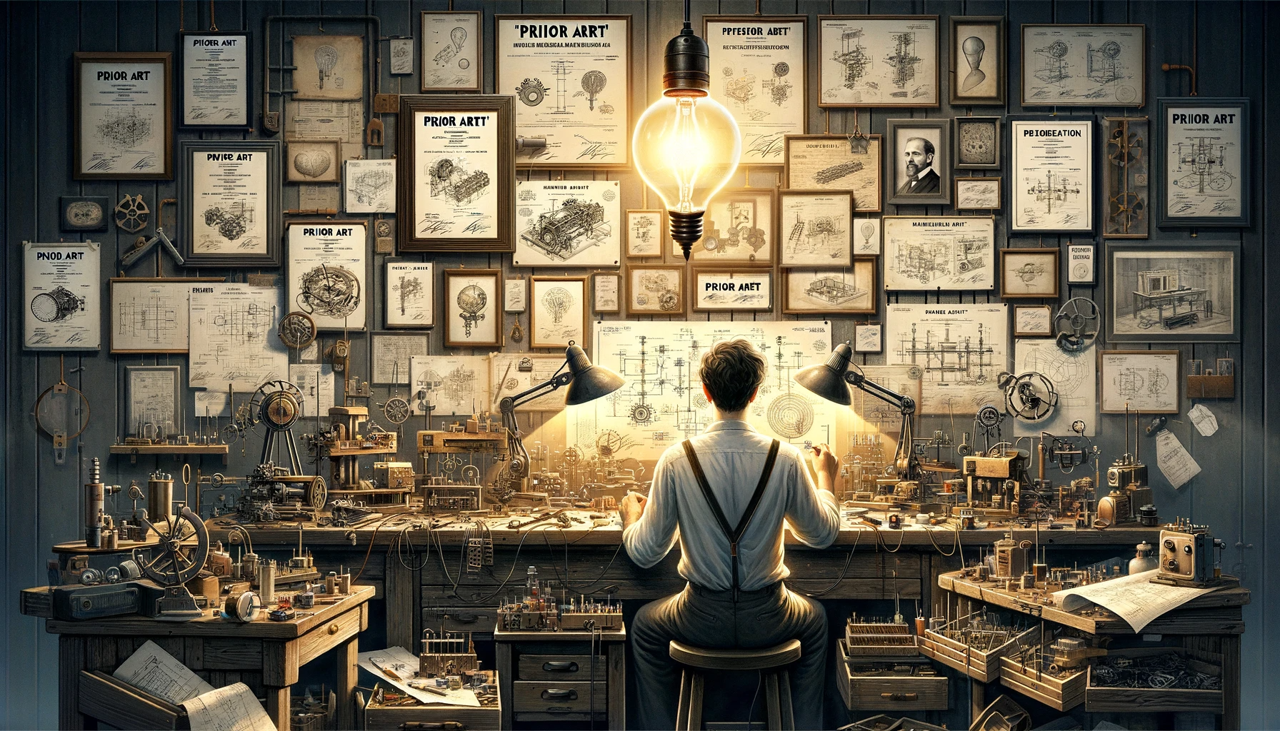In this detailed illustration, a young man sits at a large workbench in a vintage-style workshop. The background reveals vertical strips of blue-painted wood. The expansive natural wood surface of the workbench, slightly weathered to a brownish-gray tinge, dominates the scene. An additional table extends from the left in the same wood style, while another table on the right hosts numerous wooden baskets.

The man, donned in gray pants and black suspenders that form a triangular shape from his waist, sits slightly off-center to the right on a round wooden stool. He wears a neatly tucked white shirt and has short brown hair. Seated with his back towards us, he rests his left forearm on the desk while his right arm is raised as if in the midst of contemplation or work.

Surrounding him are various mechanical implements scattered across the surfaces, suggesting his role as an inventor or scientist. Two desk lamps—one on each side—provide focused illumination over his workspace. The wall behind him features a collection of framed pictures and blueprints, labeled with various spellings of "PRIORART" (e.g., PRIORARRT, PRIORARET, PRIORARTT), with each containing detailed diagrams of machines. Additional framed artworks and portraits add to the room's clutter, creating an atmosphere bustling with creativity and innovation. The intricate details of the image speak to the man's dedication to his craft amidst a setting filled with the tools and evidence of his ongoing experiments.